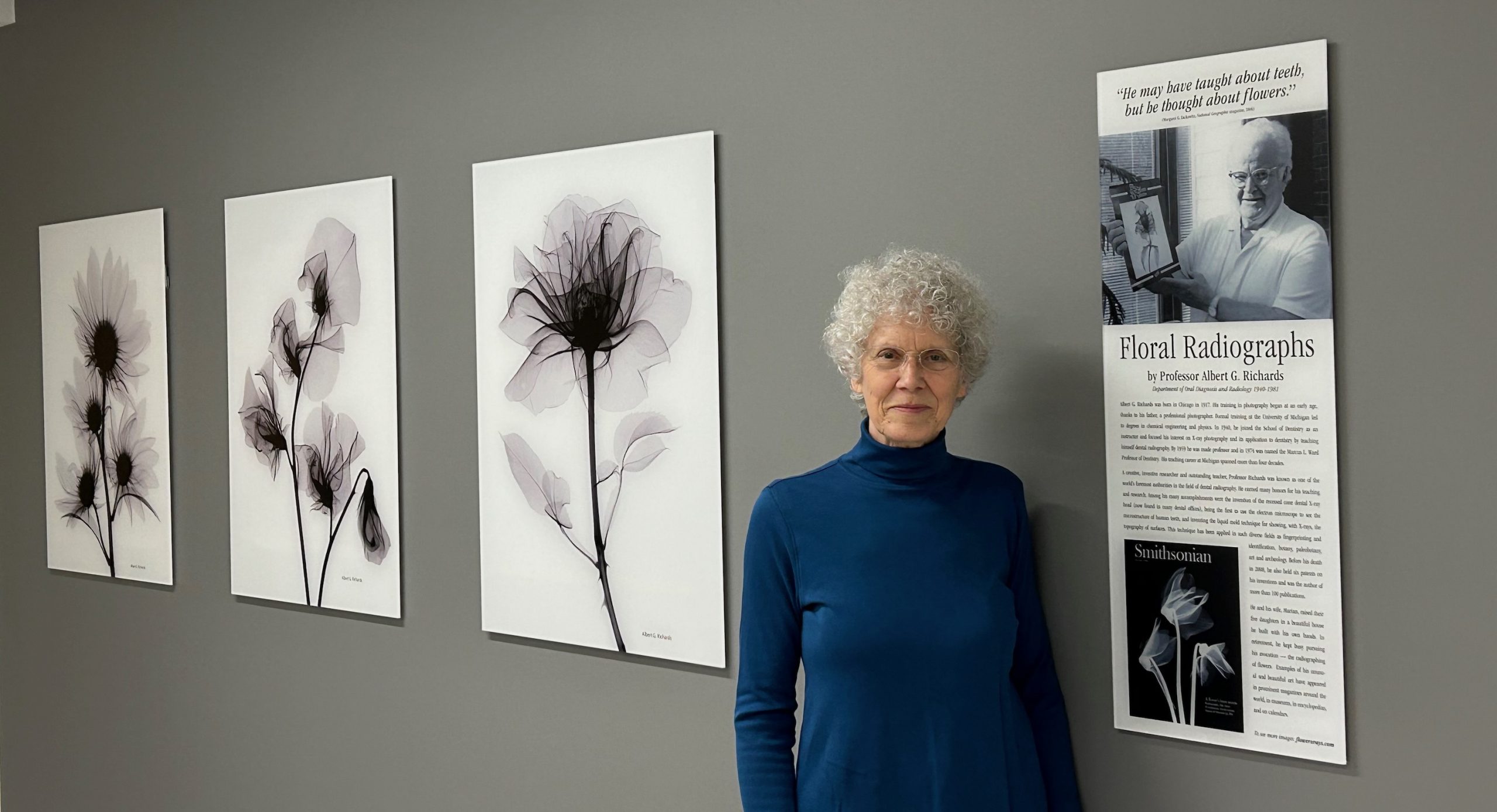The image features an older woman with short, curly gray hair, standing next to a gray wall in an art gallery. She is wearing a dark blue turtleneck and looking directly at the camera with a neutral expression, but she exudes a sense of pride. To her left, there are three black and white radiographs of flowers displayed against a white background. These radiographs, titled "Floral Radiographs by Professor Albert G. Richards," depict flowers in different states—one in full bloom, one appearing to wilt, and the last showing flowers that have completely died. To the right of the woman, a cut-out article or sign about the floral radiographs is also posted on the wall. The woman is presumably the artist, proudly presenting her work to the viewer.